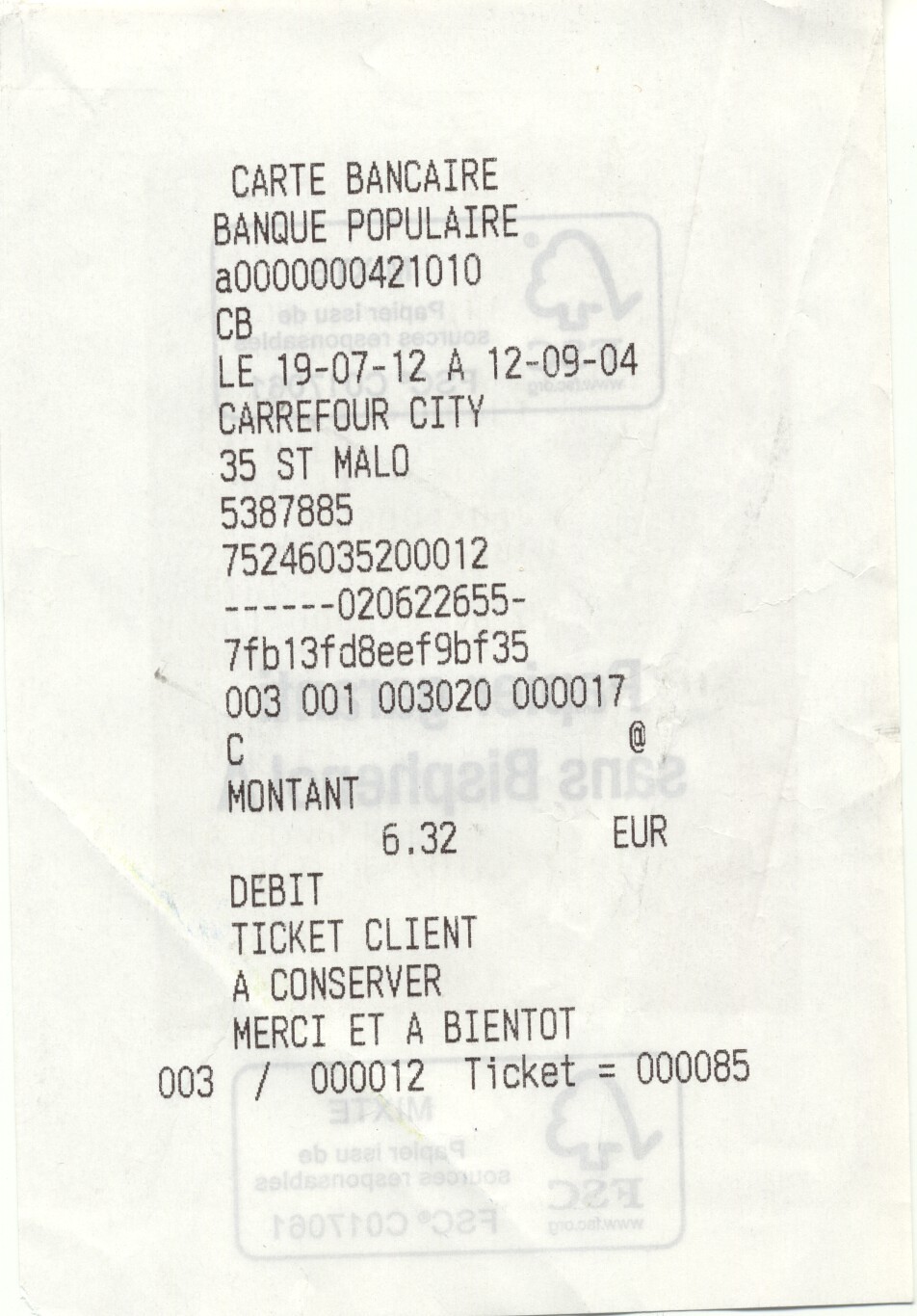The image is a black and white portrait-format photograph of a receipt, likely from a digital scan or a physical photograph. The receipt is from a financial transaction processed by Banque Populaire at a Carrefour City in Saint Malo, as indicated by the text "Carte Bancaire Banque Populaire Carrefour City, 35 St. Malo." The receipt shows a purchase amount of 6.32 euros, paid with a debit card. At the top, the term "Carte Bancaire" is prominently displayed, and lower down, "ticket client" along with various identification numbers necessary to confirm the purchase can be seen. The receipt is dated December 9th, 2004, although it might be in European format, indicating September 12th. Through the slightly translucent paper, a black outline of a stylized tree and the letters "FSC," denoting the paper's environmentally friendly status, can be faintly seen, suggesting compliance with Forestry Council standards. The receipt ends with the words "Merci" and "Bonne journée," meaning "Thank you" and "Have a good day" in French, respectively.